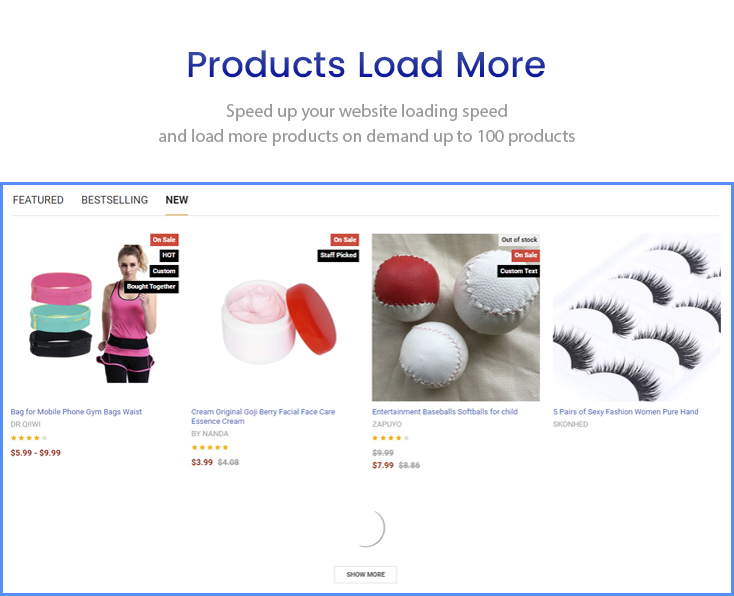The image displays a webpage interface designed for showcasing products and their loading speed. At the top, in large text, it states “Load More Products,” with a gray subtext that reads, “Speed up your website loading speed and load more products on demand up to 100 products.” This text is surrounded by a blue border box.

In the top left corner of this border, there are tabs labeled “Featured,” “Best-Selling,” and “New,” with the “New” tab being highlighted in bold and underlined. Below this, there are four product listings accompanied by images and descriptions.

1. **Bag for Mobile Phone/Gym Bag/ Waist Bag**:
   - Ratings: 4 stars
   - Price: Not specified
   - Description: An image of a girl in a pink tank top with a black belt around her waist, showing three versions of the bag in pink, blue, and black.

2. **Original Goji Berry Facial Essence Cream by Nanda**:
   - Ratings: 5 out of 5 stars
   - Price: $3.99
   - Description: A white tube with a red lid containing pink cream. It's marked as “On Sale” and “Staff Picked.”

3. **Entertainment Baseball/Softball for Child**:
   - Ratings: 4 stars
   - Price: $7.99
   - Description: Marked as out of stock.

4. **Five Pairs of Sexy Fashion Women Pure Hands**:
   - Ratings: Not specified
   - Price: Not specified

At the bottom center of the blue border box, there’s a button labeled “Show More."

The overall interface is a demonstrative representation of how rapidly a webpage can load and display multiple products, helping users visualize different product categories and details quickly.